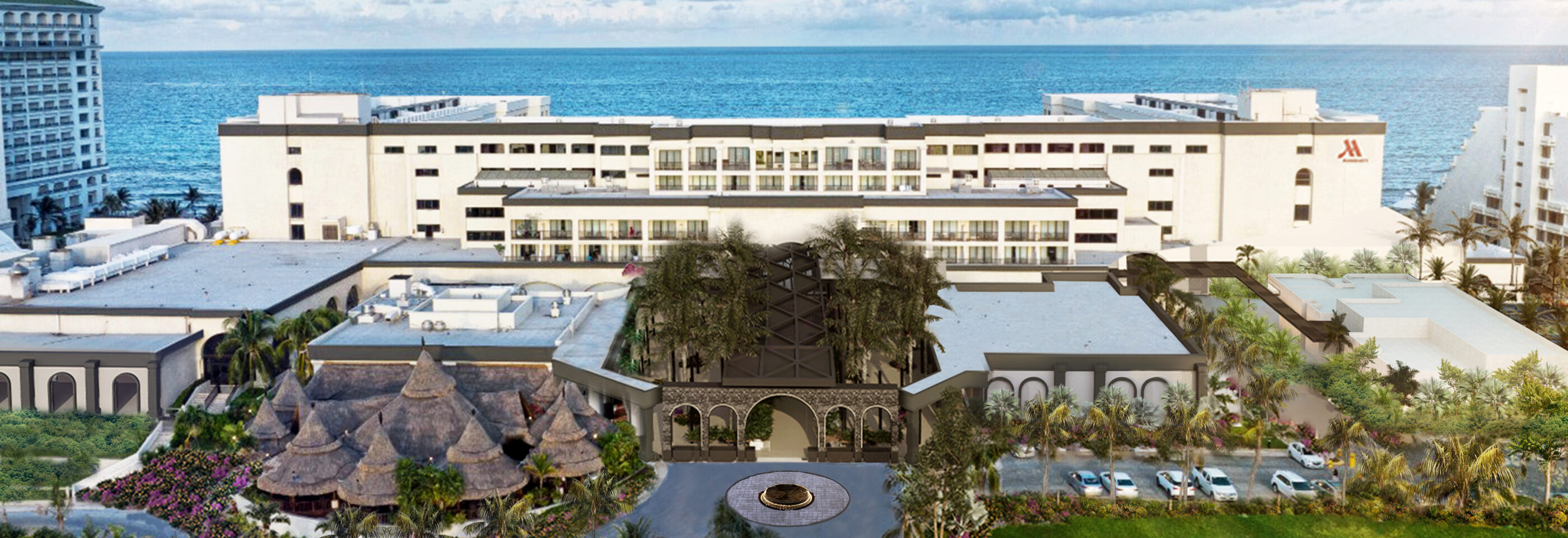An aerial photograph captures a large, five-story, white hotel situated at the edge of a seaside, likely the ocean or the Gulf of Mexico. This central building, which might be part of a Marriott chain, features numerous windows and an elaborate entrance adorned with arches and palm trees. The top right corner of the hotel displays a distinctive red 'M', hinting at its Marriott branding. To the left of the main hotel is a blue building, while to its right, there's another white building. In the foreground, there are additional smaller buildings with white rooftops, brown-tan sides, and possibly used as conference centers or related facilities. The bottom left corner of the image showcases unusual brown triangular structures resembling Aztec huts, surrounded by vibrant purple flowers and green foliage. The parking lot in front of the complex has mainly white and silver cars, with a distinct blacktop and a gray center featuring a gold element. The backdrop features a clear blue sky merging seamlessly with dark blue waters, emphasizing the hotel's beachfront location.